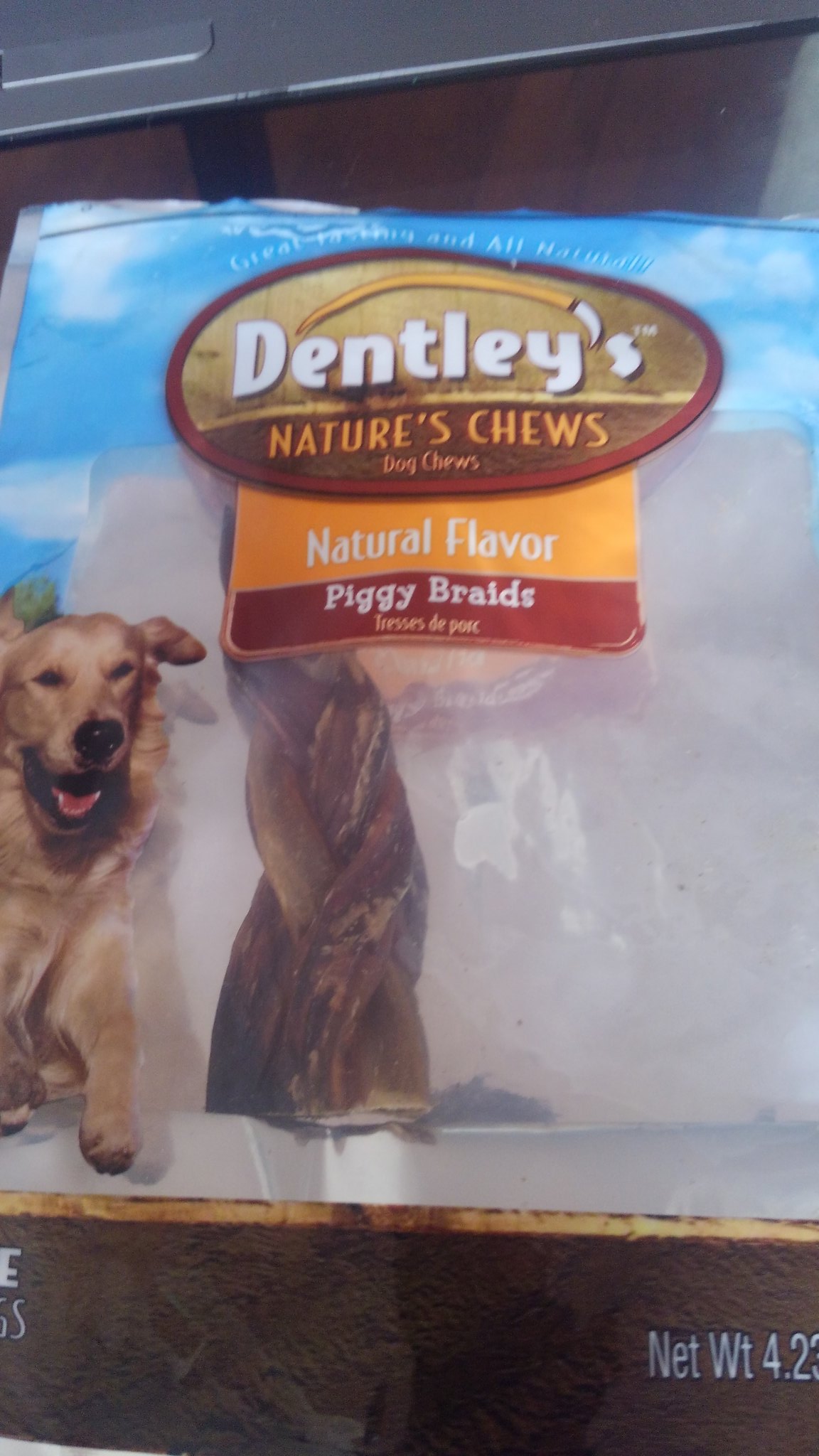The image depicts a brightly lit, clear package of Dentley's Nature's Chews Dog Treats, specifically labeled as Natural Flavor Piggy Braids. The packaging features a vibrant blue sky at the top and a black bottom. The brand name "Dentley's" is prominently displayed in white letters against a brown background at the top center, with "Nature's Chews" in orange letters underneath. Below, "Natural Flavor" and "Piggy Braids" are written in white against orange and brownish-red backgrounds respectively. 

To the left on the package, there's a vivid action shot of a happy golden retriever running. Adjacent to the dog, the treat is depicted as a braided, twisted chew. The net weight at the bottom right corner indicates 4.2 ounces, though part of it is cut off in the image. The overall scene gives a warm, natural, and inviting impression, suitable for promoting a wholesome and engaging dog treat.